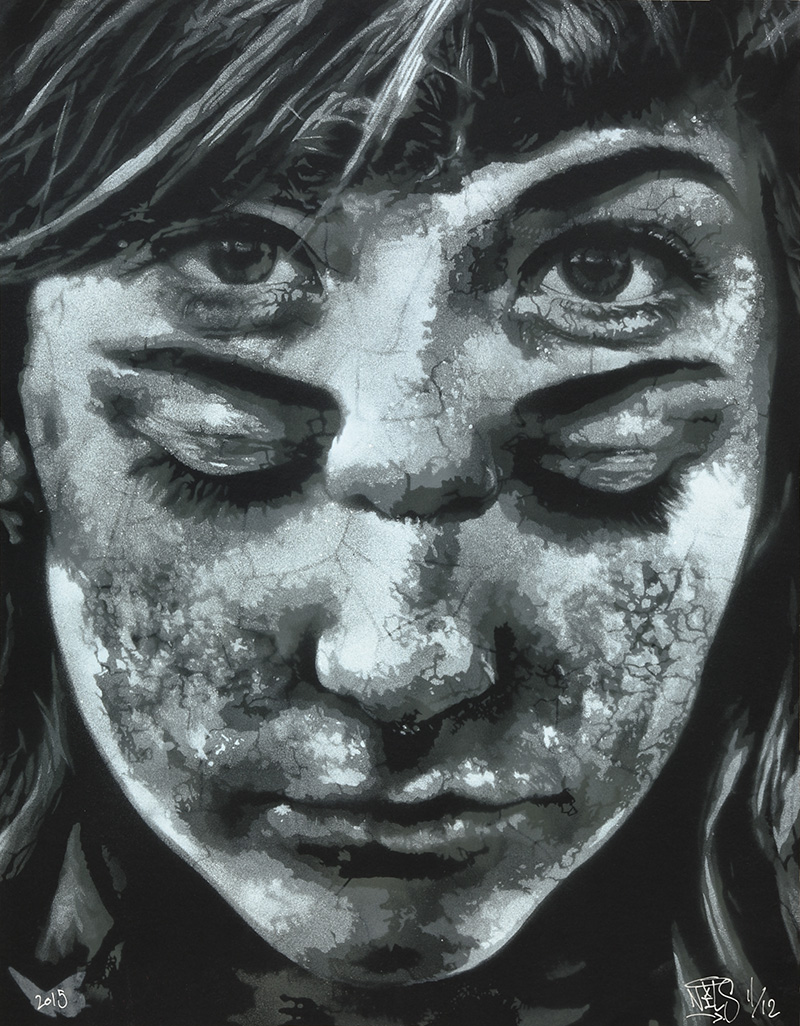This black and white painting depicts a close-up of a woman's face, rendered with a striking, cracked texture. The woman's dark hair frames her unique visage, which intriguingly features two overlaid faces. Closest to her hair is a set of eyes that are open and gazing directly forward, accompanied by a nose. Directly below, a second set of eyes are closed, with a nose beneath them. The artwork's medium appears to be a combination of paint and possibly chalk, adding to the textured look. The piece, dated 2015, includes a small signature in the lower right corner and presumably Chinese lettering. The composition suggests themes of wakefulness and sleep, with the dual faces merging into a single, enigmatic portrait.